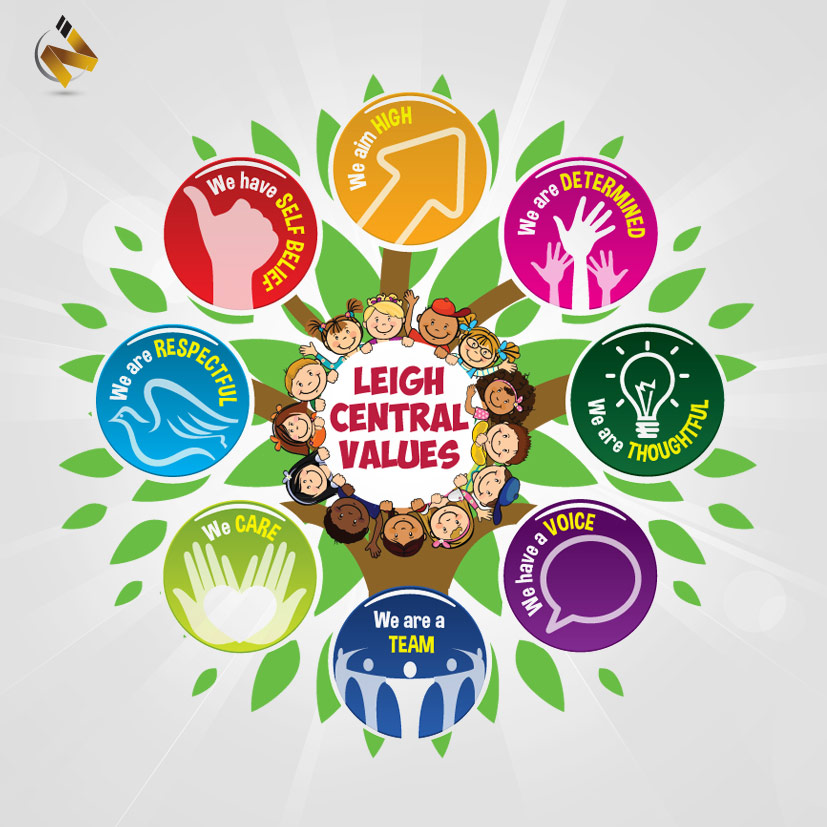The image is a detailed, vibrant illustration highlighting Lee Central Values. At the center of the graphic is a white circle with red text that reads "Lee Central Values." Surrounding this central circle are approximately a dozen animated children, each with diverse hairstyles, skin colors, and clothing, all smiling. The children are positioned uniformly around the white circle, emphasizing inclusivity and diversity.

Radiating from the central circle are brown tree branches adorned with green leaves, giving the impression of values branching out like the growth of a tree. At the ends of these branches are colorful circles, each containing a specific value and an illustration. Starting from the top and moving clockwise, the values are:

- **We Aim High** (yellow circle)
- **We Are Determined** (pink circle)
- **We Are Thoughtful** (green circle)
- **We Have a Voice** (purple circle)
- **We Are a Team** (blue circle)
- **We Care** (light green circle with a hand and heart icon)
- **We Are Respectful** (light blue circle)
- **We Have Self-Belief** (red circle with a thumbs-up icon)

In the top left corner of the image, there is an insignia resembling a ribbon with a small arc beneath it. The entire composition uses vivid colors and cheerful illustrations to create a welcoming and inclusive atmosphere.